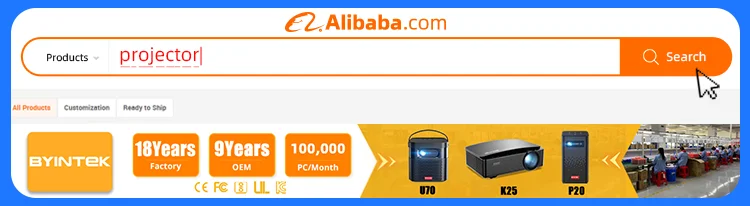In this image, we see the top section of the homepage for the website Alibaba.com. The name "Alibaba" is displayed in bold orange text, accompanied by an orange logo resembling a lowercase "n" on the left. Directly below this, there is a search bar situated on the right side, shaded in orange with the word "search" displayed in white text. On the left side of the search bar, a category selection is present which currently reads "projector" in pink text. The whole search area has an orange outline against a white background.

Beneath the search bar, there are three small tabs: "All Products" highlighted in orange on the left, "Customization" in the center, and "Ready to Ship" in black on the right. Underneath these tabs, there is a yellow (almost gold) square with white text that reads "Bintec."

To the right of this square, there are three orange squares with white lettering displaying key information: "18 years factory," "9 years OEM," and "100,000 PC/month." Moving further right, there are images of three electronic products with a gray finish set against a yellow background. Adjacent to the products, there is a glimpse of a factory section with a few people in light blue jackets working in the distance.

The entire image is bordered by a blue outline, giving it a tidy, rectangular shape.